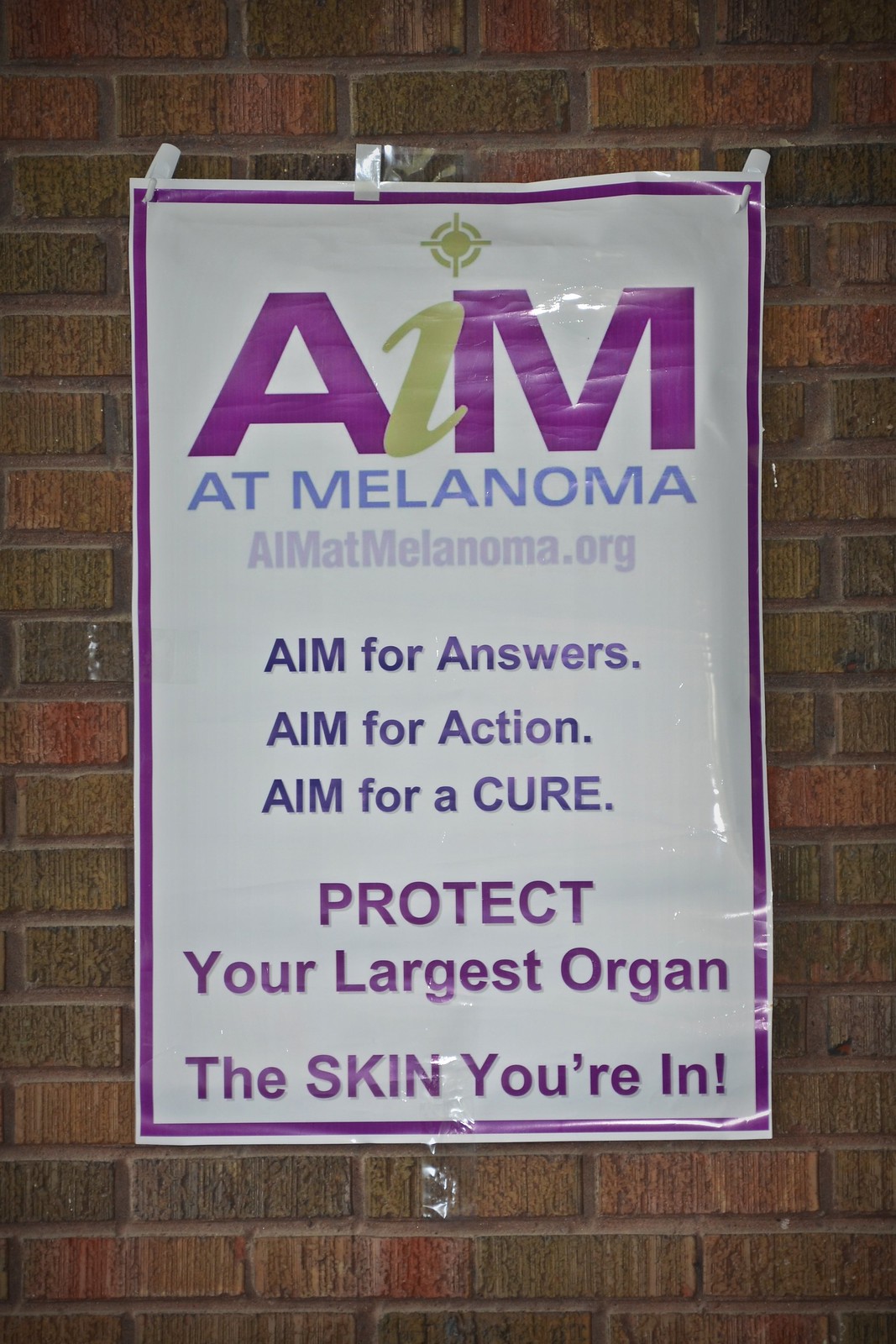This image showcases a sign affixed to a red and brown brick wall. The sign features a white background framed by a purple border. Prominently displayed at the top, the word "AIM" is written with stylistic detail: the letters "A" and "M" are purple, and the "I" is green, featuring a target symbol as the dot. Below this, the URL "AIMATMELANOMA.ORG" runs across in a light gray font. Subsequent lines in a mix of purple and light blue text read: "AIM for answers, AIM for action, AIM for a cure." Further down, in bold purple capital letters, the message stresses, "PROTECT YOUR LARGEST ORGAN, THE SKIN YOU'RE IN!" The shiny surface of the sign reflects light at the bottom, adding a visual highlight to its crisp presentation.